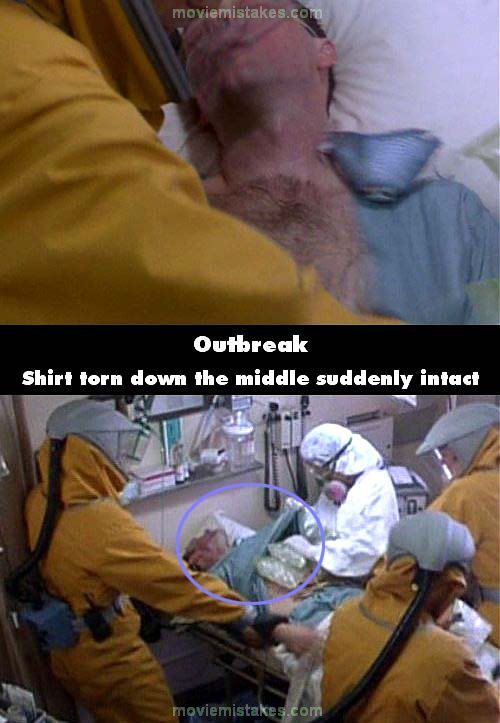A pair of sequential screenshots from the movie "Outbreak" captures a scene in a hospital emergency room. The first image shows a man with dark black hair and a torn blue shirt, lying on a white hospital bed. His hairy chest is exposed as a worker in a yellow hazmat suit tears open his shirt. In the background, a hazmat-suited shoulder is visible. In the second image, taken from a different angle in the same hospital room, the man's shirt is inexplicably intact. Surrounding him are medical staff in hazmat suits; one person in yellow is on the left while another in white places IV bags or ice packs under his shirt from the right. Additional staff in yellow hazmat suits stand at the foot of the bed. Both images feature a black band in the middle with white text that reads, "Outbreak: shirt torn down the middle, suddenly intact," highlighting the continuity error in the film, underscored by a circled area around the man's restored shirt. The source of the screenshots is identified as MovieMistakes.com.